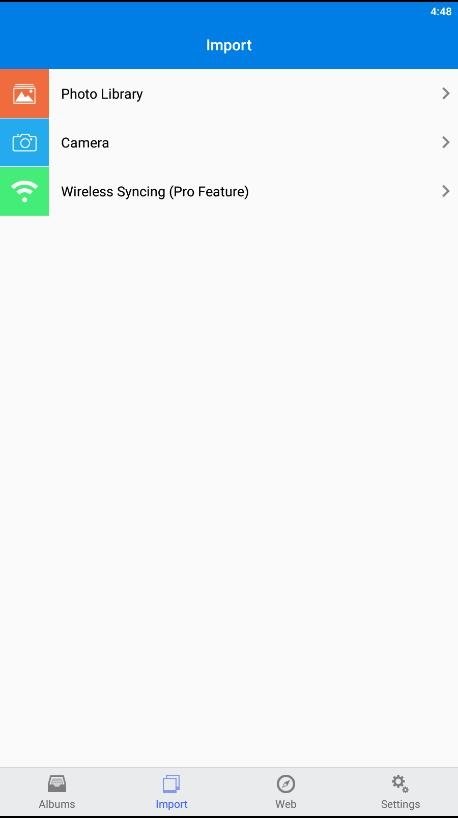This screenshot captures an interface of a photo management app on either a tablet or a smartphone. Dominating the top portion of the screen is a blue navigation bar with the word "Import" written in white text. In the top right corner, the device's time reads 4:48.

Beneath the blue navigation bar, the screen presents three options for importing photos, each accompanied by a distinctive icon. The first option, "Photo Library," is paired with an orange box featuring a photo icon. The second option, "Camera," is represented by a blue icon with a camera symbol. The third option, "Wireless Syncing (Pro feature)," is marked by a green Wi-Fi icon, indicating a premium functionality.

The app interface features a predominantly white background. At the very bottom of the screen, four tab options are available for navigation. These include:
1. Albums
2. Import (highlighted in blue, indicating the current active page)
3. Web
4. Settings

This organized layout facilitates easy access to different sections of the app for managing and sharing photos.